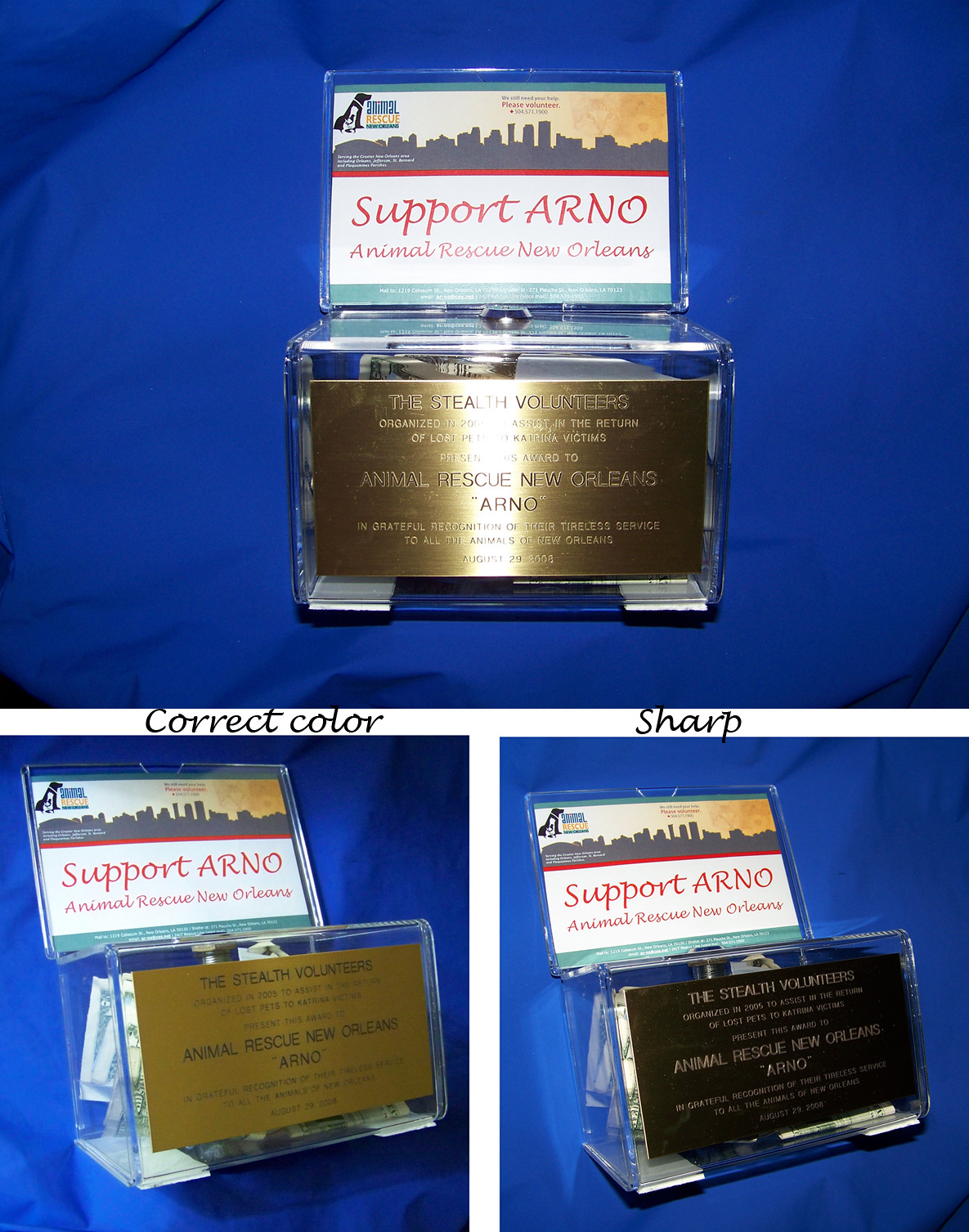The image showcases three clear donation boxes resting on a bright blue cloth. Each box features a gold-plated plaque in the center, engraved with "The Stealth Volunteer" and "Animal Rescue New Orleans (ARNO)." The plaque is housed within a plastic container and is flanked by two metal rods, one to the left and one to the bottom right, providing support. The primary image of the box is mirrored in two smaller images positioned at the bottom left and right, each offering different angles. The bottom left image includes text that reads "Correct Color" at the top, while the bottom right image features the word "Sharp" in cursive. Above the plaque, a colorful card displays "Support ARNO" in script lettering alongside an illustration of the New Orleans skyline, framed by a blue and orange sky. Inside one of the boxes, visible dollar bills indicate money that has already been donated. The entire arrangement appears staged for the photograph, with no additional elements in the background.